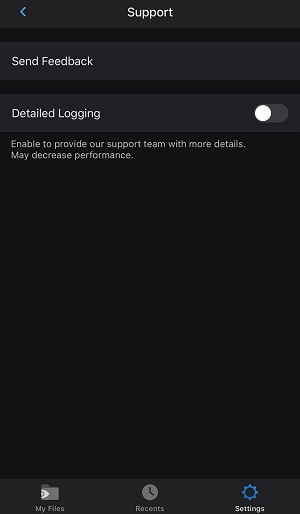The image features a smartphone screen displaying the "Settings" page, with a focus on seeking support. At the top of the screen, the word "Support" is prominently displayed, signaling the user's intent to find assistance. Below this title, there are two distinct options: "Send Feedback" and "Detailed Logging."

The "Send Feedback" option can be selected, as indicated by a tappable button, though no visual slider is associated with it. The "Detailed Logging" option features a slider button currently positioned to the left, indicating it is turned off. Beneath the "Detailed Logging" option, there is a cautionary note stating that an inability to provide the support team with detailed logs may decrease performance.

At the bottom of the screen, three navigation icons are visible against a slightly lighter black background. These icons represent different functions: the one related to "Settings" is highlighted in blue, depicted by a gearbox symbol. Alongside it are icons for "Recent" activities and "My Files."

Additionally, the top left corner of the "Support" page features a blue arrow, which signifies the option to navigate back to the previous screen. The overall background of the screen is black, with the text and icons primarily in contrasting shades for better visibility.